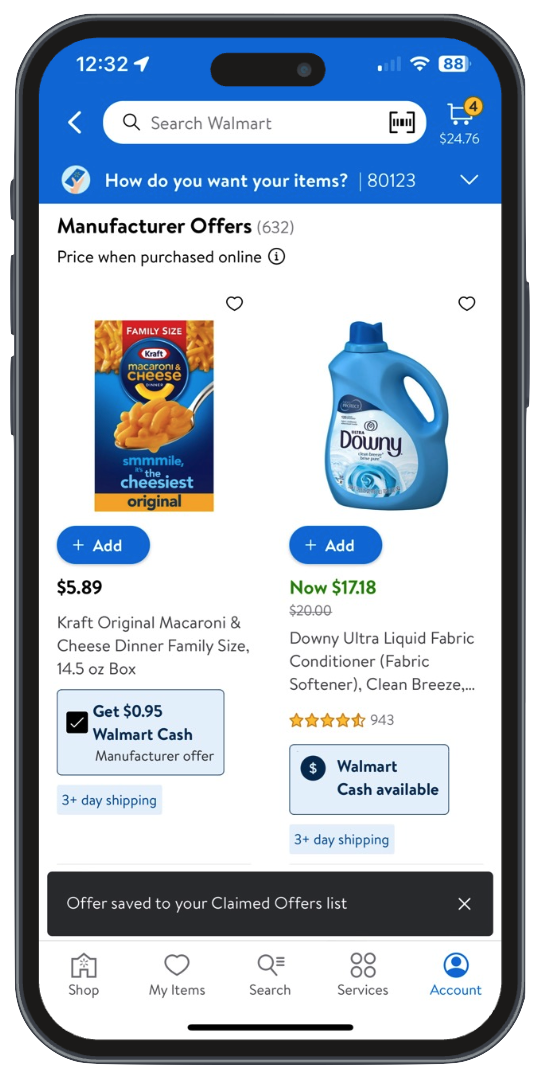The image depicts a smartphone displaying the Walmart app on the home screen, showing the time as 12:32. At the top of the app interface, there is a back arrow for navigation and a search bar for Walmart. Adjacent to the search bar is a button for a barcode scanner. The cart icon indicates that the user has four items totaling $24.78. Below, the app prompts "How do you want your items?" and mentions the zip code 80123. This specific page focuses on manufacturer offers, highlighting that there are 632 available.

The first visible offer is a family-sized box of Kraft Original Macaroni and Cheese Dinner (14.5 oz), priced at $5.89. The product includes an option to add it to the cart with a blue “Add” button and indicates that purchasing it would earn $0.95 in Walmart cash as a manufacturer offer. This item also offers three-day shipping.

Next, the image shows Downy Ultra Liquid Fabric Conditioner Fabric Softener Clean Breeze, priced at $17.18. This product also features the blue "Add" button. It has nearly four and a half stars based on 943 ratings. The product is accompanied by a dollar sign indicating Walmart cash availability and mentions an offer being saved to the user's claim offer list, along with three-day shipping available.